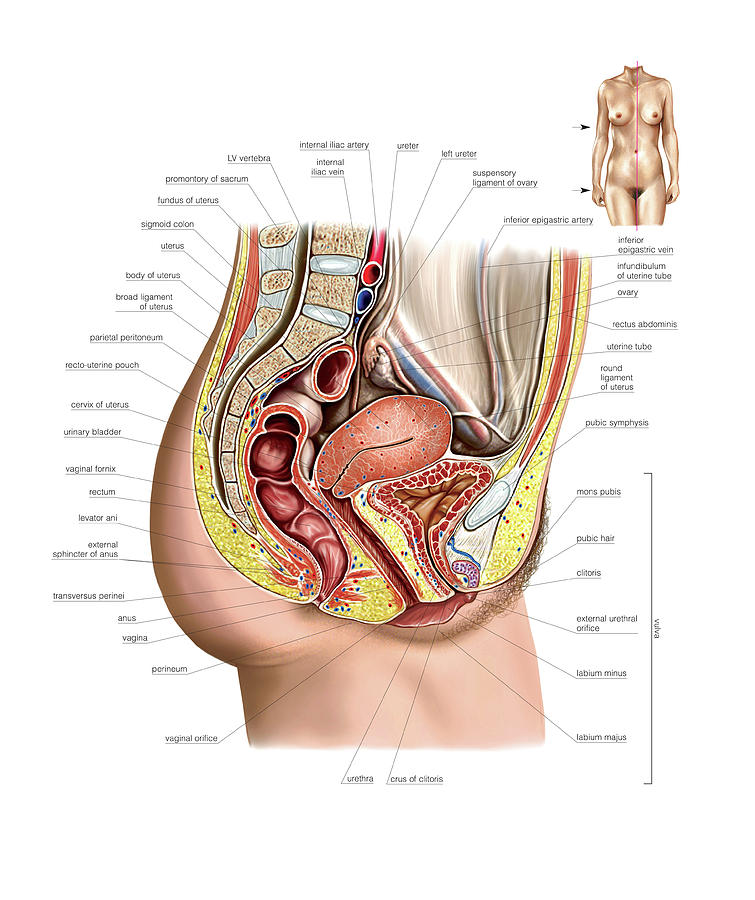The image is a detailed anatomical illustration of a woman's lower body, focusing on the pelvic and abdominal regions. In the top right corner, there is a smaller inset showing a frontal view of a female body from the thighs down, confirming the subject's gender. The main image is a side view cross-section revealing the internal structures, including the spinal cord, lower spine, intestines, and major blood vessels situated in front of the spine. It also details various vital organs in the pelvis, such as the ovaries, uterus, and vaginal area, complete with extensive labeling—approximately 40 labels—pointing to different parts of the anatomy. Arrows and lines extend from these labels, clearly identifying each specific organ and structure, providing a comprehensive visual study of the lower female anatomy.